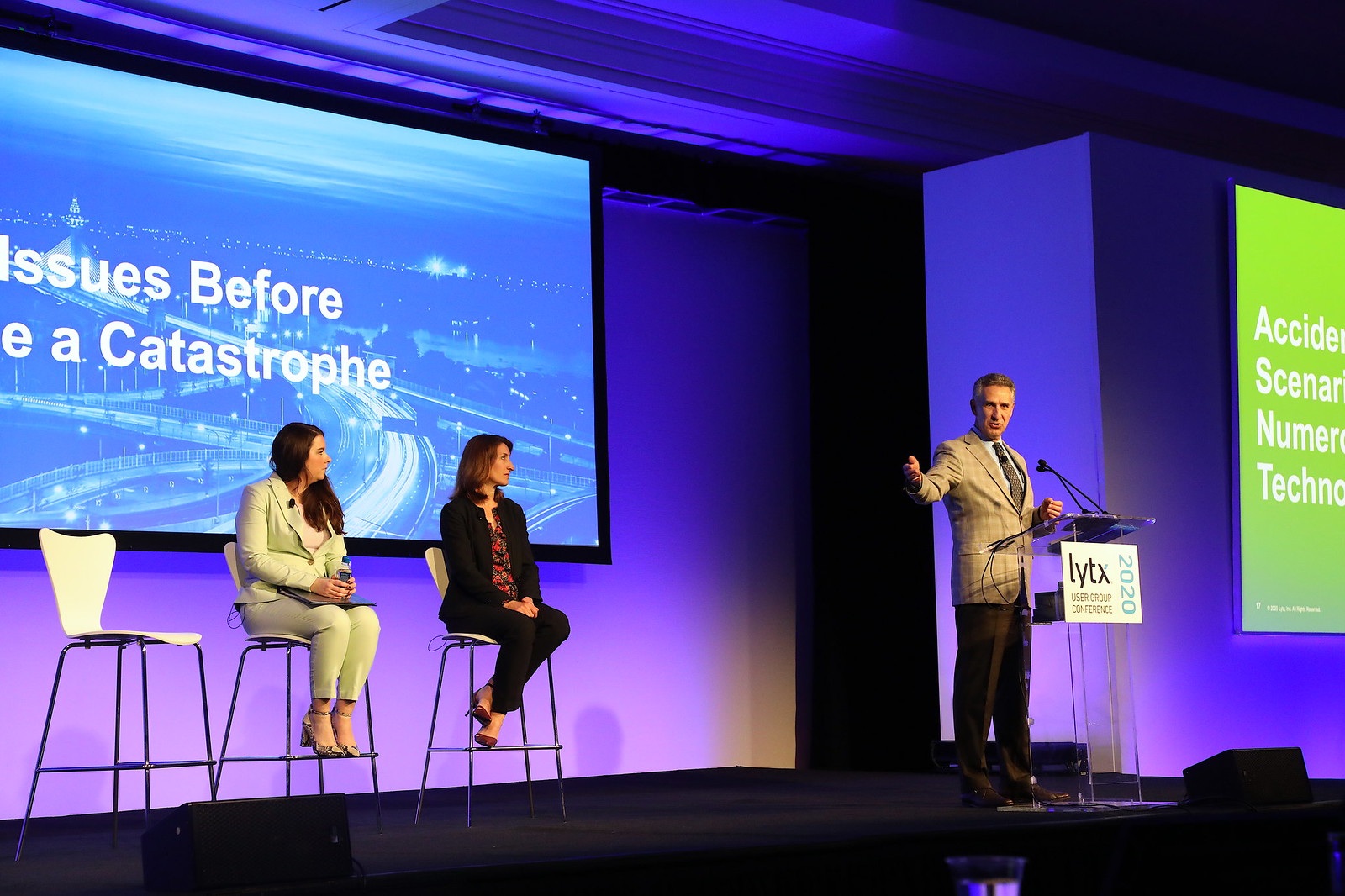A detailed image depicts a dynamic event setting on a stage with distinct elements and characters. At the center, an older man stands confidently behind a clear podium that displays the sign "LYTX User Group Conference 2020." He is dressed in a beige plaid jacket with a dark brown tie and contrasting dark pants. His hair is streaked with gray, and he appears to be in mid-speech, stretching his right arm outwards and engaging with the audience. The stage backdrop is a dark purple wall transitioning to a lighter purple hue at the bottom. 

Behind the man, there are multiple screens reinforcing the visual layout of the stage. One prominent screen says "Issues before a Catastrophe," possibly displaying an image of a city, although partially obscured. Another smaller screen, positioned to the speaker's left (audience's right), is green and reads "Accident," though the full text is unclear.

Flanking the man on stage are three white high chairs. Two of these chairs are occupied by women who are attentively focused on the speaker. The woman on the far right, with short brown hair, is dressed in a mostly black attire paired with a red and black t-shirt under a black sweater and high heels. The woman seated next to her has longer brown hair and wears a pale green outfit. The empty chair to their left completes the seating arrangement. The visual ambiance is further enhanced by the rich purple lighting that bathes the stage, creating a professional yet engaging atmosphere.